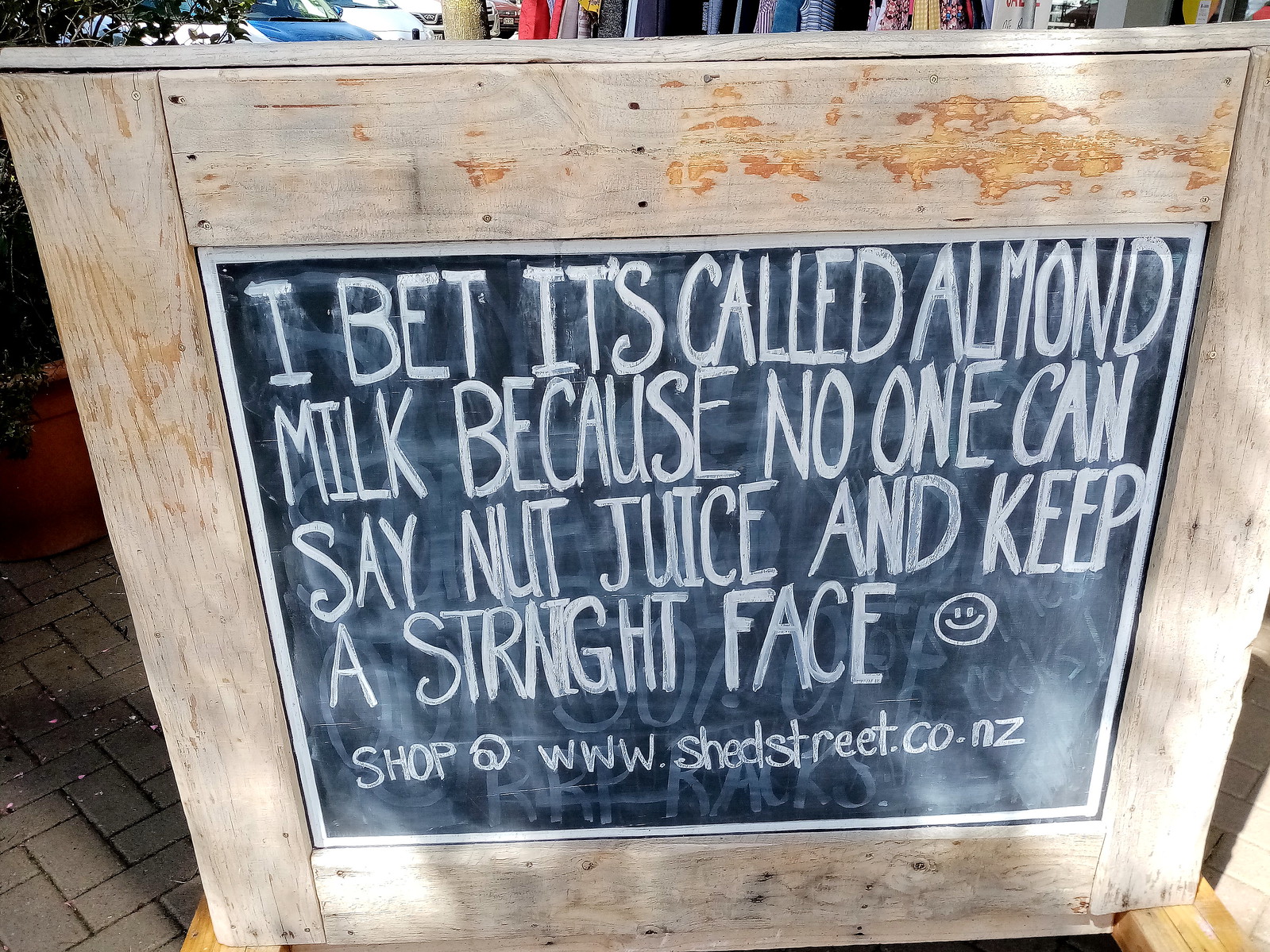The image shows a chalkboard sign surrounded by a wooden frame that appears to be slightly peeling and rusting, revealing orangish-brown patches. The sign is positioned on a brick floor, likely at an outdoor or semi-outdoor cafe. The chalkboard, with legible, broad white letters, reads: "I bet it's called almond milk because no one can say nut juice and keep a straight face." Beside this text is a smiley face emoji. Below, in a smaller font, it reads: "shop at www.shedstreet.co.nz." In the background, blurred hints of cars and possibly people add to the outdoor setting. The detailed rustic look of the wooden frame highlights the casual, inviting atmosphere of the cafe, suggesting it may be a quaint spot in New Zealand.